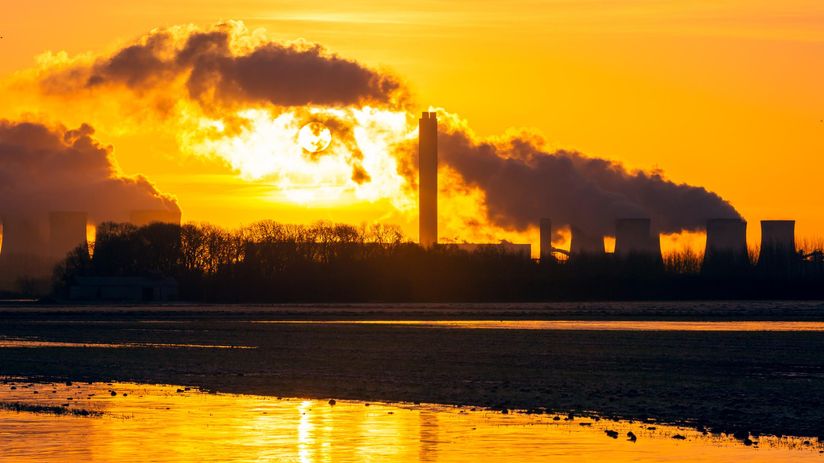The image is a rectangular, realistic photograph taken outdoors during sunrise or sunset, casting an orange, reddish, and yellow hue across the sky, which contains both the sun and the moon. Dominating the center is an industrial factory setting, featuring a tall, thin smokestack emitting smoke against the colorful backdrop. To the back left, there are curved towers, akin to those at a nuclear power plant, also releasing vapor. Dark silhouettes of trees are visible against the vibrant sky. The foreground shows a field and a small body of water, possibly a puddle or river, reflecting both the industrial structures and the glowing, warm colors of the sky. The scene is both striking and somber, highlighting the interplay between industrial elements and natural beauty.